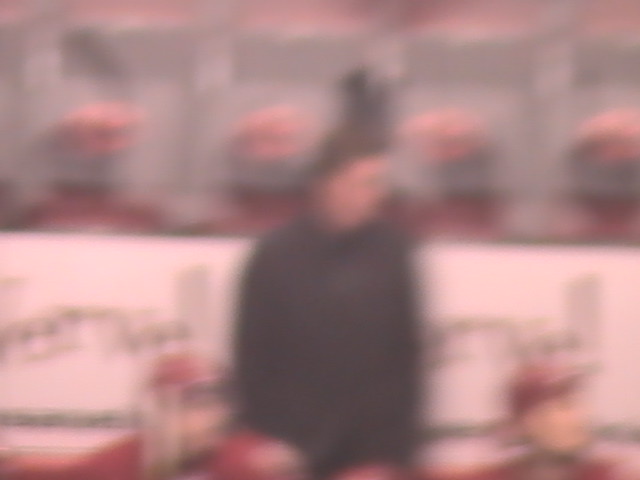The image is a very blurry depiction centered around a person, possibly a woman, standing against a backdrop that appears to be a white barrier with some black writing on it. The person's long dark hair is styled upwards, and they are wearing a dark long-sleeve shirt and dark pants. The individual's facial features are indistinguishable, though their head is slightly turned to the right. 

Above the white barrier in the background, there are four objects with a reddish circular shape, possibly windows or lights, adding a fairground or amusement park-like ambiance with a lot of pink and red hues. Below these objects, there appear to be figures, possibly paintings or mannequins, dressed in red baseball caps and red shirts. These figures are positioned on either side of the central person, with their faces also turned to the right. The figures add a sense of symmetry to the image, though the overall scene remains indistinct due to the poor focus of the photograph.